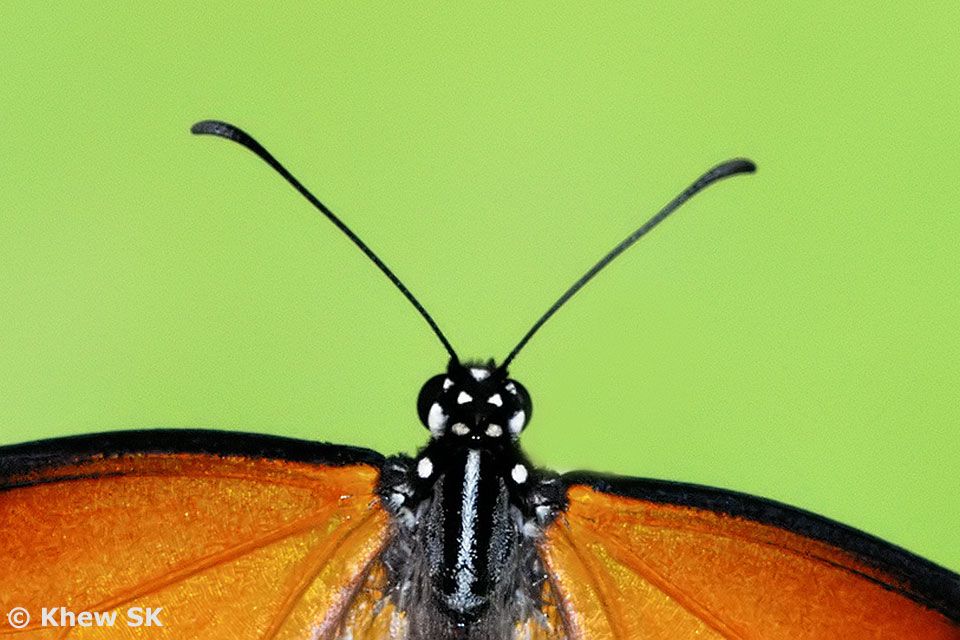This is a highly detailed close-up image of a butterfly set against a vivid lime green background, which occupies about 75% of the photograph. The butterfly is positioned in the lower portion of the image, seemingly moving from the bottom to the top. This striking insect features a black head adorned with white spots, two long, narrow antennas extending to each side, and protruding eyes. The black body is covered in fine white fur with a distinct white stripe running down its back, adding to the texture and fuzziness visible in the photograph. The wings of the butterfly are a vibrant orange, transitioning from a darker shade near the edges to a lighter hue towards the center. They are outlined with a bold black border, and the intricate veins are distinctly visible, giving them a shiny appearance. The detailed depiction of both the butterfly's body and wings provides a lifelike impression, almost resembling a highly detailed drawing or painting. Copyright QSK, KHEW, SK.